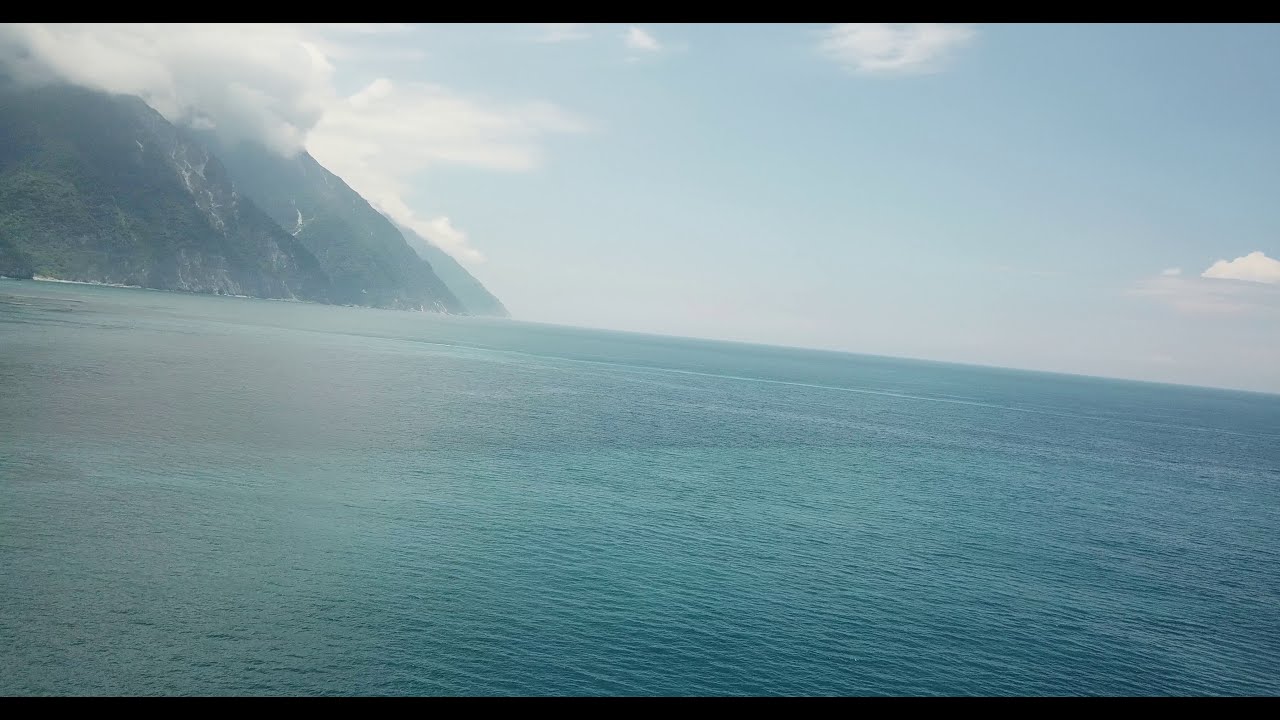The photograph captures a vast, serene ocean with a striking greenish-blue hue, extending from the foreground to the horizon. The camera is slightly tilted to the right, adding a subtle diagonal slant to the composition. On the left side, the ocean meets imposing rocky cliffs and tall hills, which are enveloped by lush greenery. These landforms rise steeply from the water, their summits shrouded in puffy, white clouds that merge with delicate fog descending the cliffs. The sky above is a light blue, dotted with a few scattered clouds, with the denser, larger cloud formations concentrated above the hills. Despite the brightness of the scene, the sun is not visible. The landscape is unmarred by human presence or activity, with no people, ships, or text to distract from nature’s tranquility. The predominant colors are the vibrant green-blue of the ocean, the soft light blue of the sky, and the darker, earthy tones of the hills and cliffs.